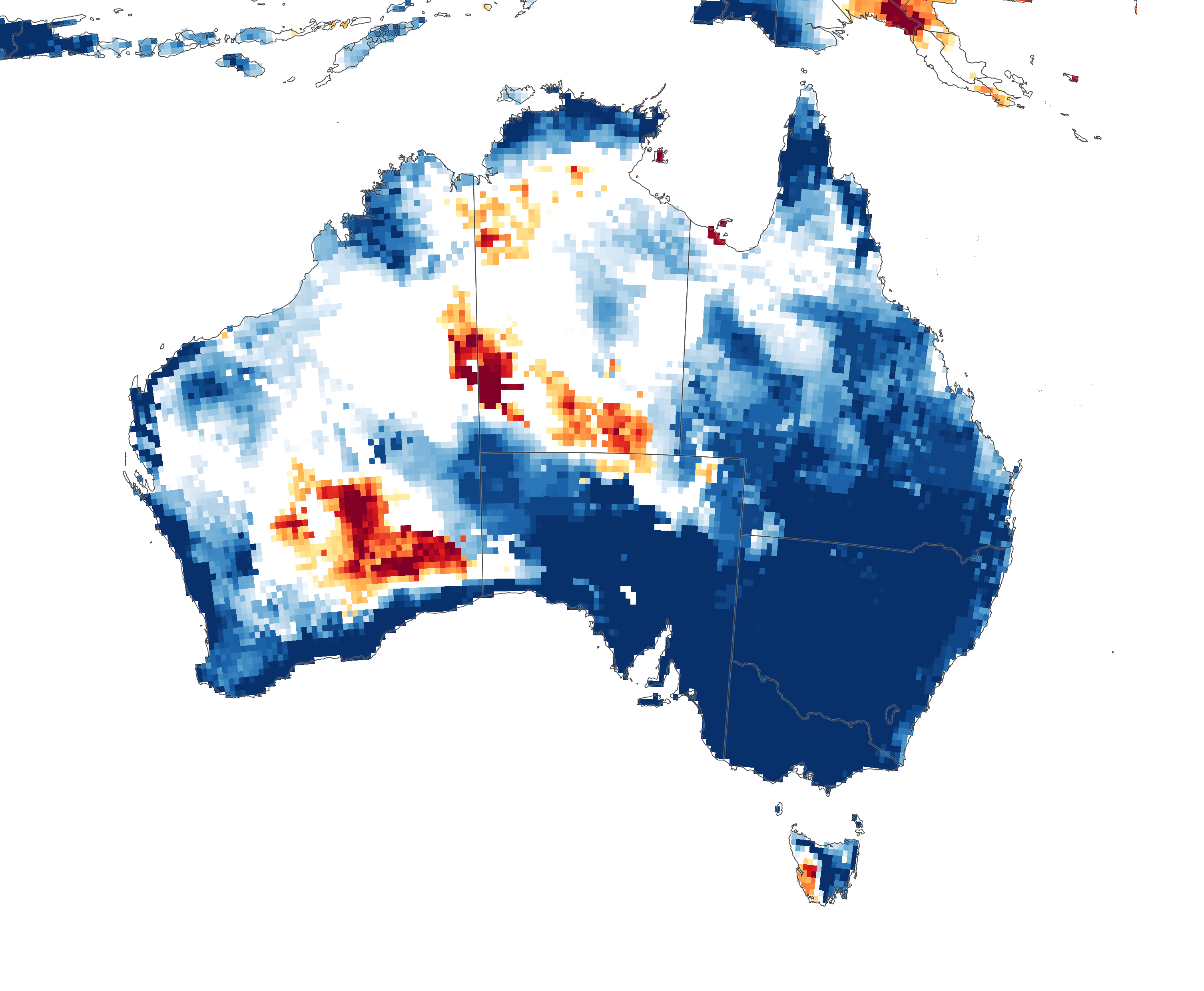The image in question is a detailed map of Australia, pixelated to represent the terrain with distinct colors. The ocean surrounding the continent has been removed, creating a cut-out effect similar to clip art. You can also see parts of other continents above Australia. The map features a range of colors, including dark blues, light blues, whites, reds, oranges, and browns, which indicate various elevations. The majority of the dark blue colors are concentrated in the lower right-hand corner of the map. Thin black lines segment the map into different regions, resembling an old TV's pixelation with tiny squares composing the surface. The overall image appears somewhat fuzzy and blurry, and it gives an impression of a weather map based on how the colors are distributed.